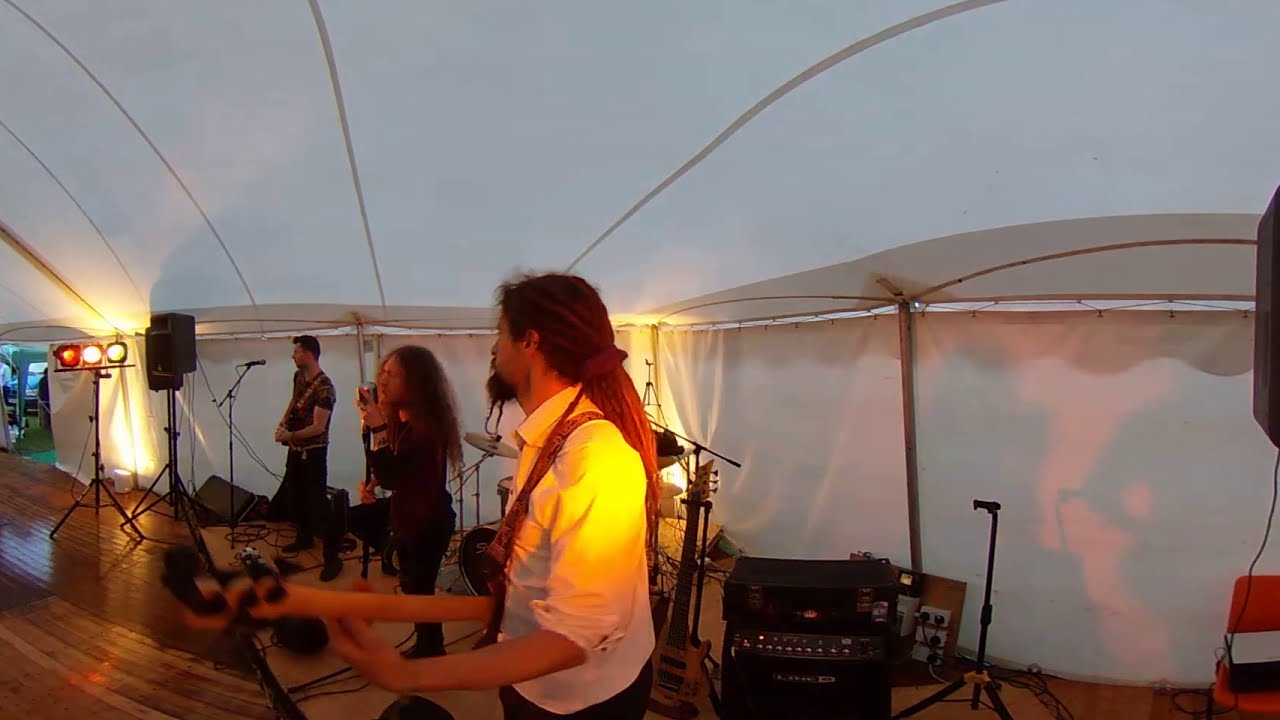This is a detailed image of a band performing under a large white tent, possibly at a church gathering or a wedding reception. The setting is indoors with a photographic style as the scene is lit by artificial lighting. In the foreground, a white male musician with long dreadlocks tied back and a braided goatee is seen wearing a white button-down shirt. He appears to be playing a bass guitar. To his right, a woman with long, curly brown hair dressed in black is singing into a microphone. Her figure is partly obscured by the other performers. Further right, another musician with long hair, unstyled, also dressed in black, is singing into a microphone. In the background, there is a fourth man with a short haircut, wearing a short-sleeved shirt and dark pants, who appears to be playing a guitar while singing into a microphone. The scene is surrounded by various musical equipment, including speakers on stands, wires, cables, and lights. Part of a drum set is visible behind the band, although the drummer himself is obscured. The performers are standing on a hardwood floor, and a floating chair is visible in the bottom right-hand corner of the image. There is no text on the image.